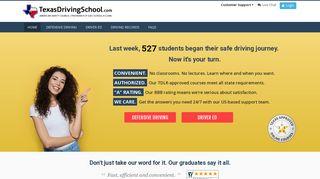The image depicts a website for the Texas Driving School, characterized by a low resolution that makes detailed reading difficult. The header of the website is set against a white background, with "Texas Driving School" prominently displayed on the left side. Adjacent to it on the right side is a blue button with the text "Log In" in white. Directly beneath this is a dark blue or black horizontal strip featuring five links, though their text is illegible due to the poor quality of the image.

The main section of the webpage has a yellow background, with a photograph of a woman situated on the left side. She is pointing towards the right side of the screen. Accompanying the image is a caption: "Last week, 527 students began their safe driving journey. Now it's your turn. Convenient, authoritizing...," the ending words are unclear but imply a message of encouragement and convenience.

Below this text are two red buttons with white text, although the exact wording is indiscernible. In the bottom right corner of the yellow section is a round emblem featuring a yellow star at its center, surrounded by text that follows the circular shape; however, the specific content of the text remains unreadable.

Below this yellow rectangle, the description provided does not continue. The poorly rendered image makes detailed interpretation of further elements impossible.